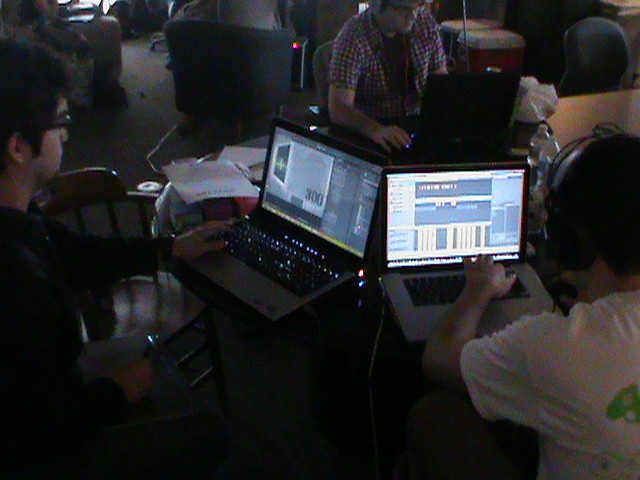The photograph captures a dimly lit room where three young Caucasian men in their early 20s are seated around a circular brown table, each engrossed in their laptops. The room, which resembles a darkened living room or an internet cafe, features a beige carpet and a couch in the background, adding to its cozy yet cluttered atmosphere. 

On the left, a young man dressed in black with dark hair and glasses is intensely focused on his laptop, which displays a screen filled with settings and details, possibly indicating an editing program. In the middle, directly across from the viewer, sits another young man in a white and red flannel shirt; his laptop's screen is not visible to the camera. On the right, a third young man, wearing a white t-shirt with a blue logo on the back and a headset, is also engrossed in a program on his laptop, which appears to involve audio mixing or some sort of console interface, with noticeable numbers and controls visible.

Scattered on the table are various items, including pieces of paper, a bottle, and some tissue, hinting at a prolonged period of focused work. All three men are wearing glasses and headphones, fully immersed in their respective tasks, adding to the scene's overall atmosphere of concentrated effort in a shadowy, intimate setting.